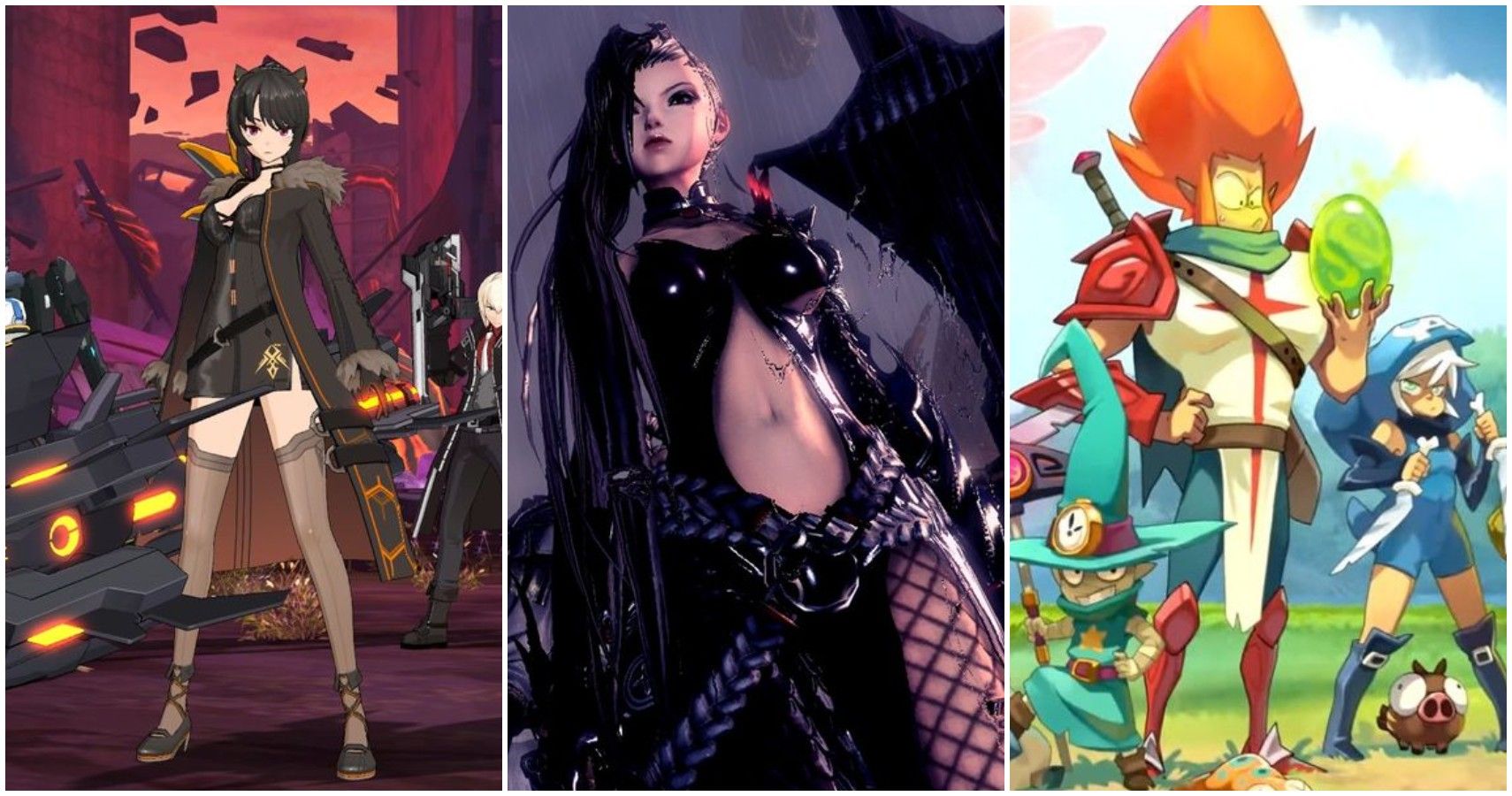The image is segmented into three distinct cartoon-themed scenes. The left section features an anime-styled woman set against a futuristic, dystopian backdrop. She dons a revealing outfit with a brown fur coat, tie stockings, and high-heeled boots. The backdrop includes a ship resembling an orange-lit futuristic motorcycle and a male figure with a high-tech gun. The middle section showcases another dark, dystopian scene with a female video game character. She has a partially shaved head, long hair cascading from the other half, and is clad in a tight black corset and fishnet leggings. The atmosphere is ominous with pouring rain and a looming dark tower. The right section shifts to a vibrant, cartoony setting, featuring a male character with exaggerated, flaming red hair, dressed in a medieval-style outfit complete with a red shoulder pad, red boots, and a sword hilt. He holds a green egg, and beside him stands a girl in a skin-tight blue outfit with white hair, wielding white bone-like daggers. Additionally, a small wizard with a green hat adorned with a clock and a matching robe holds a wand. A small, brown pig with large eyes and a pink nose is also present, heightening the whimsical feel of this segment.